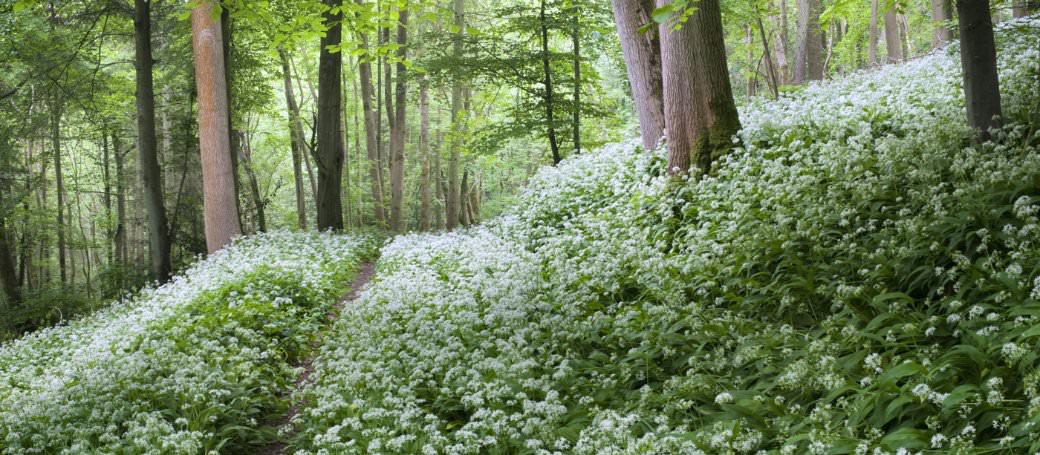This detailed landscape photograph captures a serene and vibrant forest meadow. The image, which is wider than it is tall, clearly depicts a dense canopy of green foliage interspersed with numerous slender trees that resemble aspens. The trees have brown trunks, varying from thick to fairly skinny, forming a scattered and lush wooded area. The forest floor in the foreground is densely covered with green plants and foliage. Amongst this verdant carpet, there are thousands of scattered white wildflowers, creating a striking contrast against the green. The image conveys a bright and clear day with abundant natural sunlight, enhancing the vividness of the greens and whites. There are no animals, humans, words, or numbers present, allowing the natural beauty of the outdoor setting to be the sole focus.